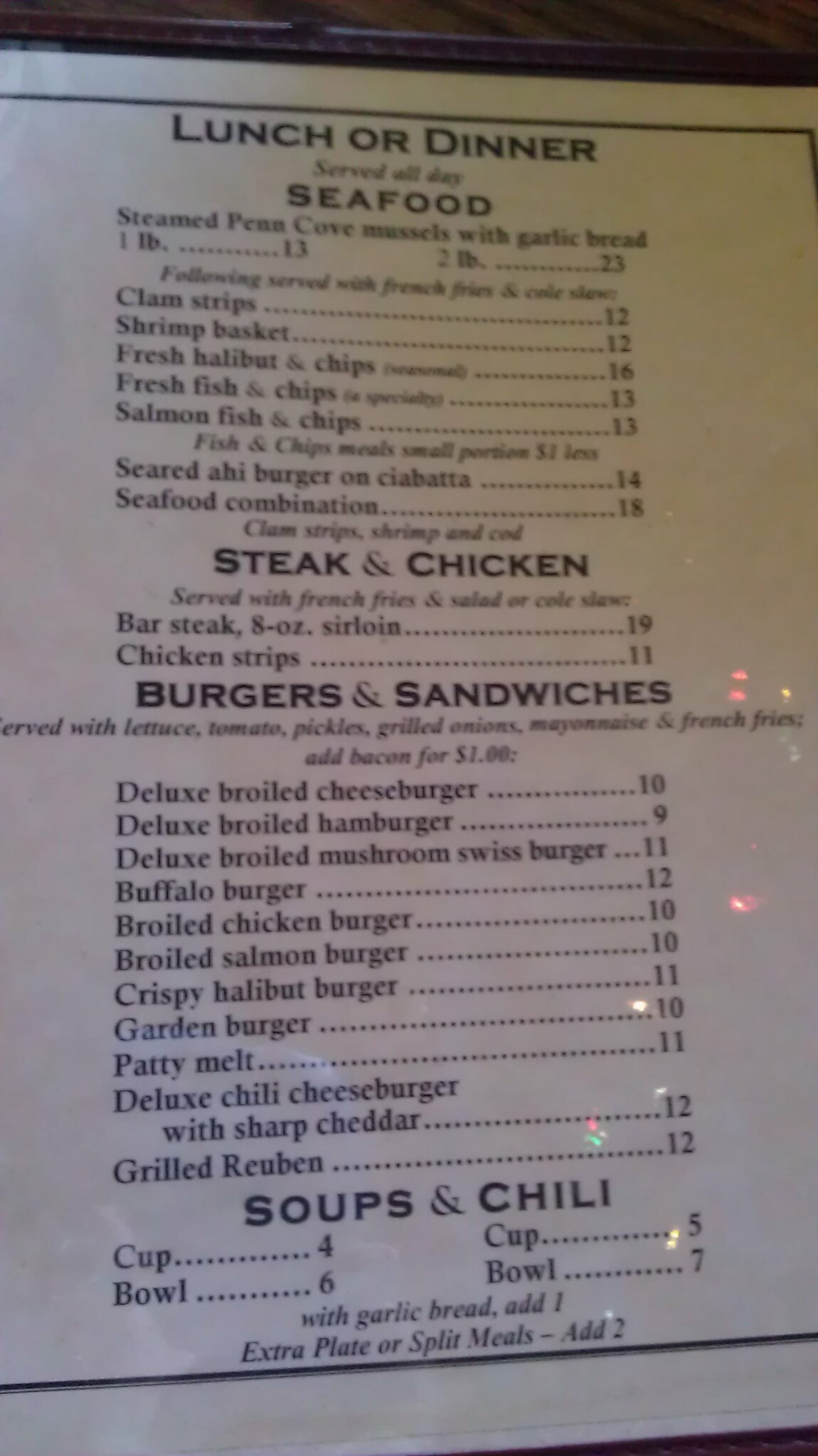The colour photograph captures a detailed image of a dining establishment's menu encased within a dark brown menu holder, photographed at a slight angle from the top, which reveals the holder's horizontal edge at the top of the image. The menu itself appears to be laminated or covered in plastic, resulting in numerous light reflections on the lower half of the menu, especially towards the right-hand side where the reflections exhibit red, white, and green hues. Despite the image being slightly soft in focus, the text remains legible.

The menu features bold, black text in various sizes. At the top, it prominently states "Lunch or Dinner Served All Day" followed by "Seafood." The menu is divided into sections: "Steak & Chicken," "Burgers & Sandwiches," and "Soups & Chilli," with ampersands used in place of "and."

Specific menu items listed under "Seafood" include "Steamed Penne Cuvée" with mussels and garlic bread, "Clam Strips," "Shrimp Basket," and "Fresh Halibut and Chips." Each item is followed by a dotted line leading to a price on the right side of the menu. Although slightly blurred, the organizational structure and textual elements of the menu are clear and structured for easy reading.